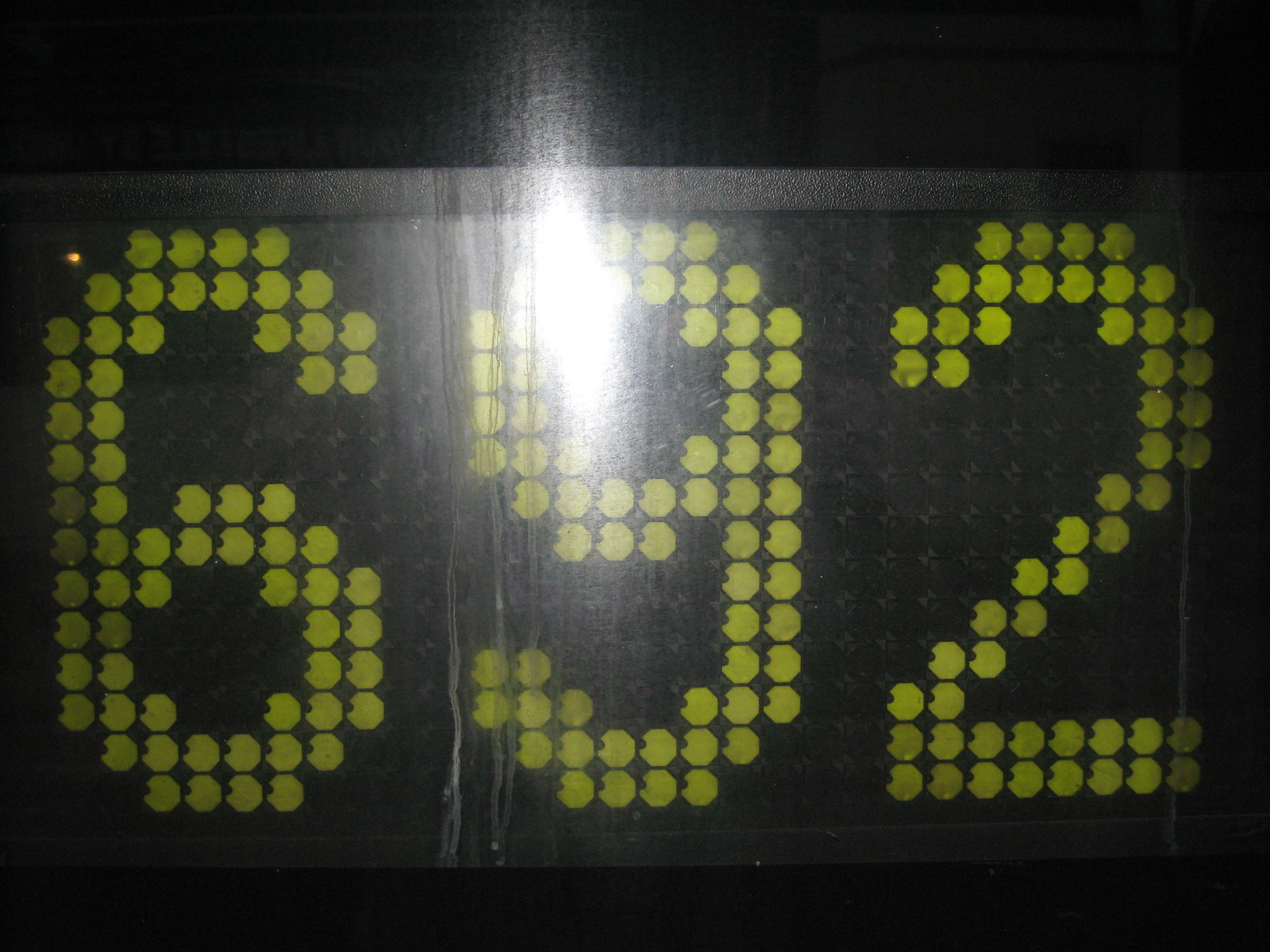This close-up image features a black platform displaying three numerals in a greenish-yellow hue. The unique design of the numerals resembles Pac-Man characters, each with a slight opening on the left side. From left to right, the numbers are '6', '9', and '2'. Notably, a splash of white light illuminates the top part of the '9', adding a striking contrast. The background surrounding these numerals is a uniform black, with the top and bottom sections of the image showcasing an even darker shade, further emphasizing the luminous greenish-yellow digits.